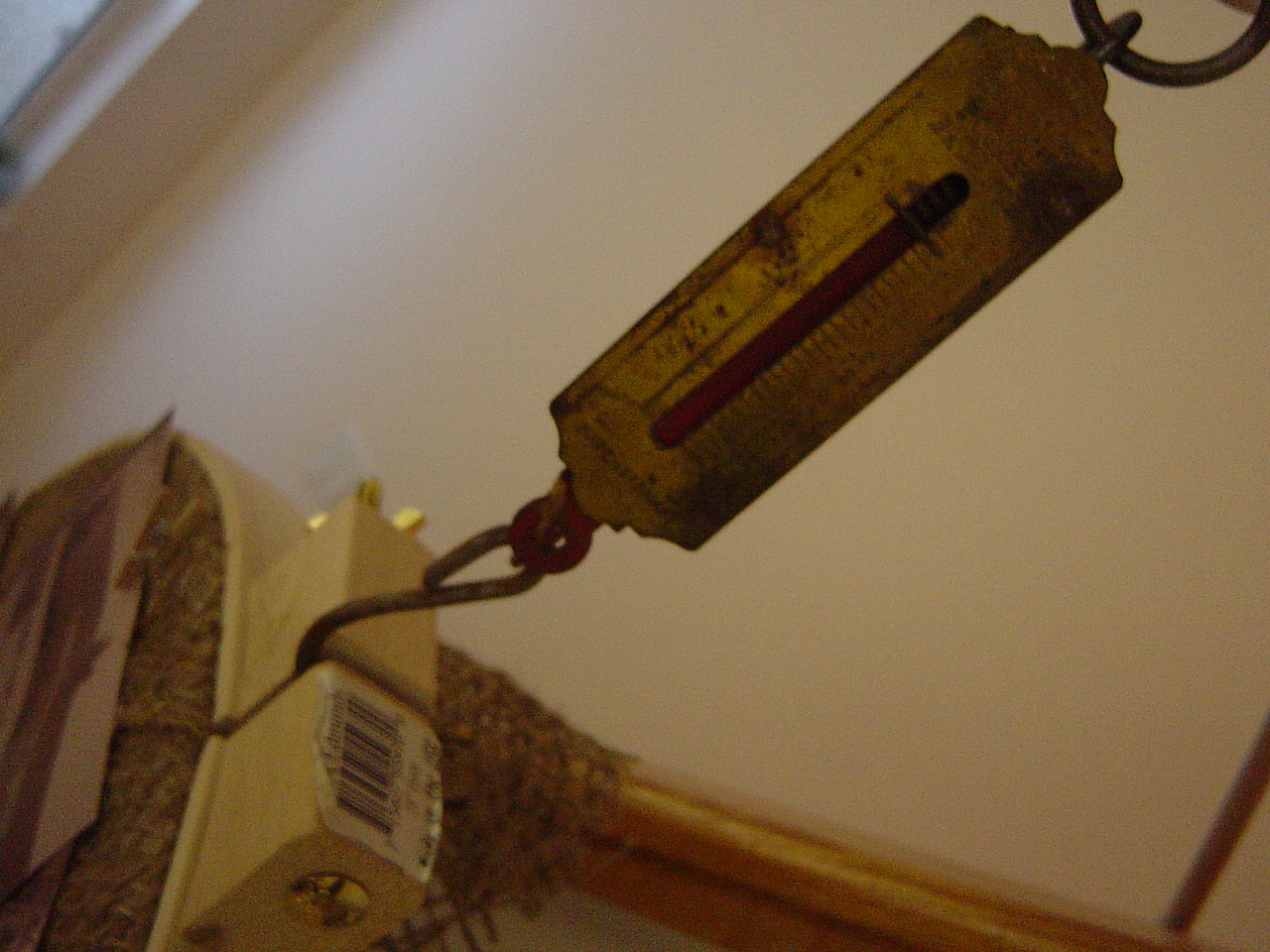A close-up image reveals a grimy, stone-like object with a rough rectangular shape and irregular top and bottom edges. Attached to this object is a circular, red component at the bottom, which is connected to a metal hook. This hook appears to be squeezed by two white, beige-colored pieces, possibly part of a clamp mechanism. The background features a white wall, though the exact nature of the objects remains unclear due to the proximity of the shot.